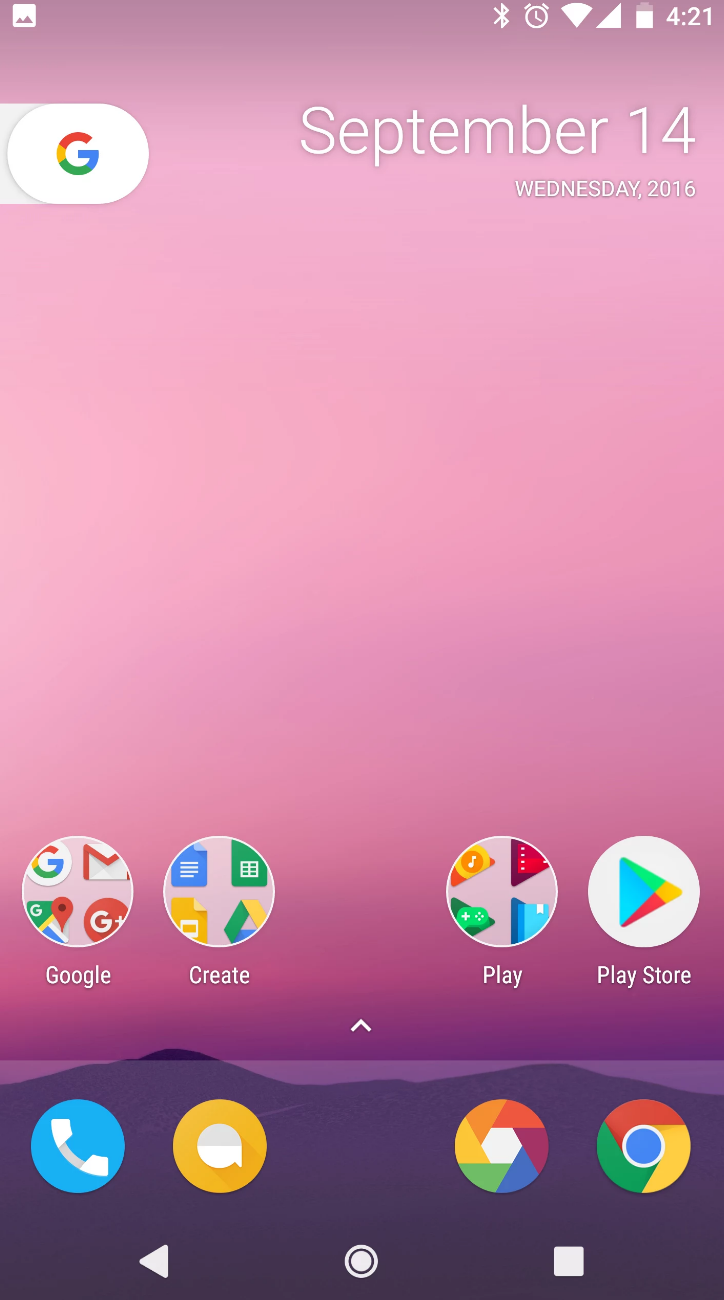In this image, we are presented with a colorful screenshot of a phone's home screen. The background transitions from a vibrant pink at the top to a soothing lavender as it moves downward. In the upper left corner, the gallery icon is visible, while the upper right corner displays the status icons including Wi-Fi signal, the clock showing 4:21, and the date, "September 14th, Wednesday 2016," in white text.

On the left side of the screen, a white box contains the "G" from Google. Towards the bottom section of the screen, we observe four circular folders organized neatly, each encompassing a set of apps. The first folder, labeled "Google," includes apps such as Gmail and Google Maps. The second folder is labeled "Create," followed by the third folder named "Play," and finally the fourth folder titled "Play Store."

At the very bottom of the image, there are several app icons displayed in circles. From left to right, there is a telephone icon in a blue circle, an orange circle with a white central dot, a circle with the multicolored Google "G," and finally the Google Chrome browser icon, which features the colors green, red, yellow, and blue.